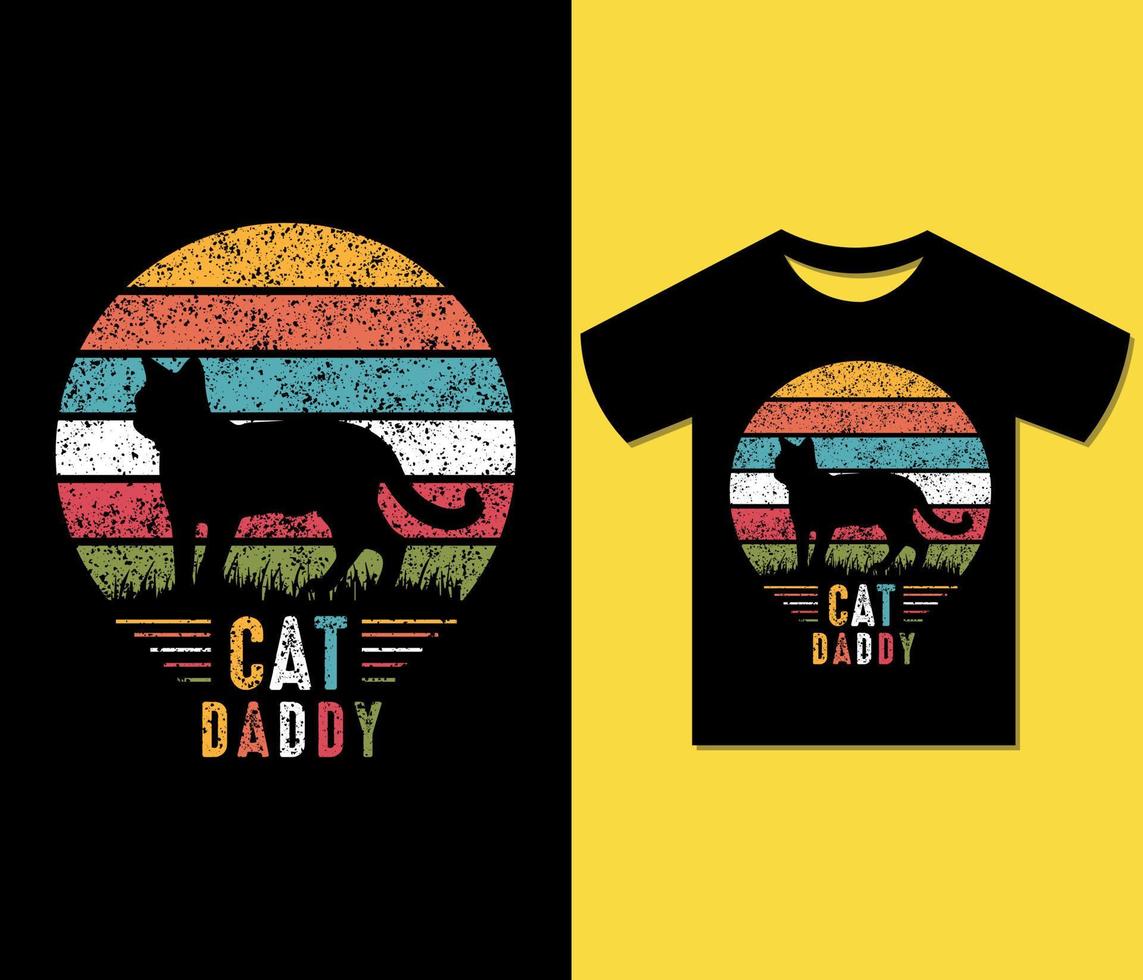This image features a side-by-side view of a t-shirt and its graphic design, providing a clear and detailed representation of both. The left side showcases the standalone graphic set against a black background. The decal highlights the phrase "CAT DADDY" in a variety of colorful letters, including shades of yellow, white, teal, orange, green, and red. Above the text, multicolored stripes—orange, pink, blue, white, red, and green—form a circular pattern, within which a solid black silhouette of a cat walks on black grass. On the right side, the black t-shirt with the same vibrant decal is displayed against a yellow background, emphasizing how the design appears when printed on the shirt. The overall presentation is visually appealing but does not provide any information regarding the designer or purchasing details.